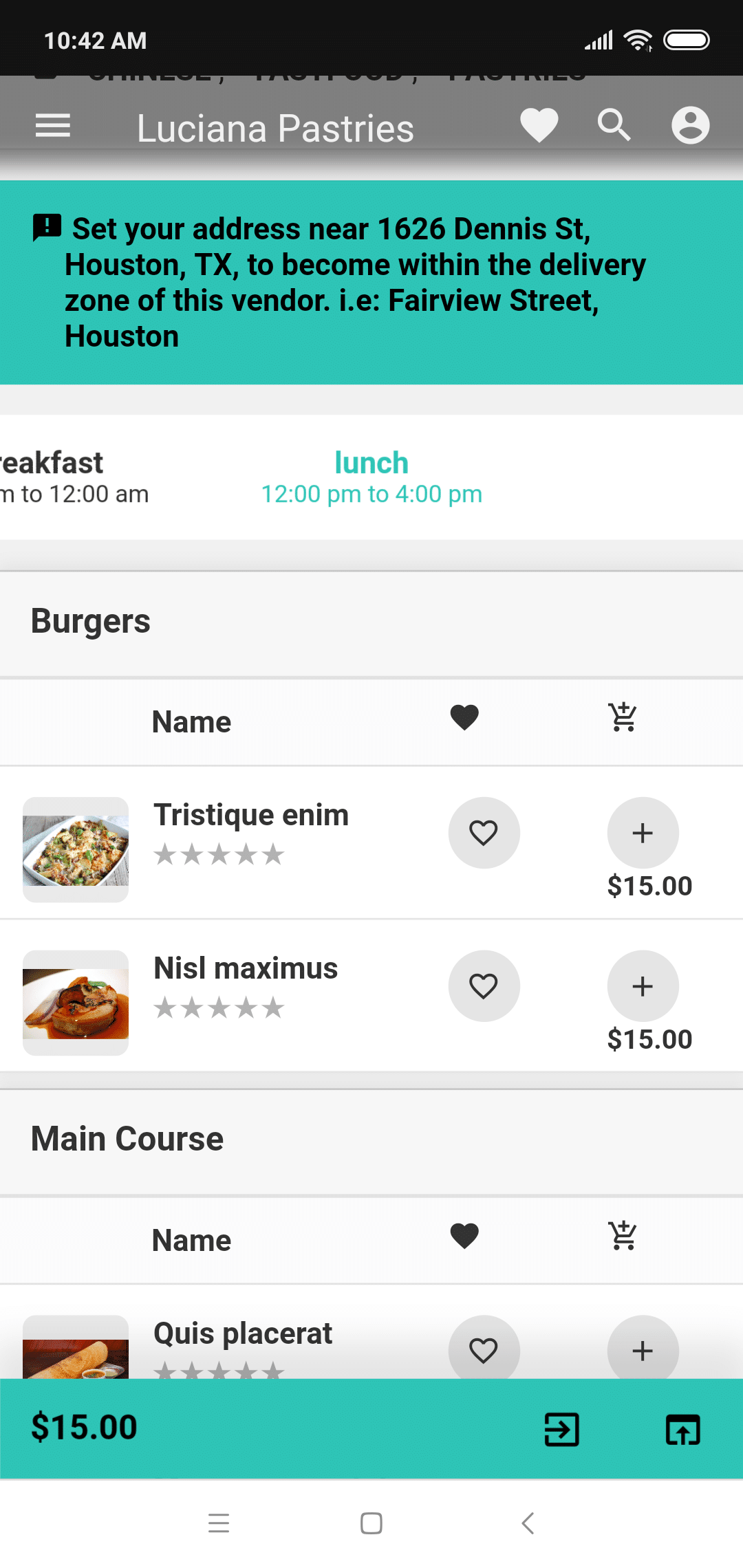A detailed description of the image shows a food delivery service interface, potentially from an app like Grubhub or DoorDash. At the very top, a black status bar includes standard cell phone icons: the time "10:42 AM" is displayed on the left, and on the right, full indicators for battery, Wi-Fi, and cellular reception are shown in white.

Below the status bar, the majority of the screen is a white background, framed by teal blue bars at both the top and bottom. The bottom bar displays a running total of $15. Above, the top bar prompts the user to "Set Your Address" and provides details about delivery proximity to the selected vendor.

The vendor, "Luciana Pastries," is highlighted just below the black status bar, with white text on a gray background. Interface icons, including a hamburger menu to the left, favorite heart, search, and profile icons, are also present.

The time of day is 10:42 AM, and the app indicates that Luciana Pastries serves lunch from 12 PM to 4 PM. The user is browsing the lunch menu, specifically looking at burgers and main courses. There are a few options listed, each priced at $15, although the menu items are in an unfamiliar language.